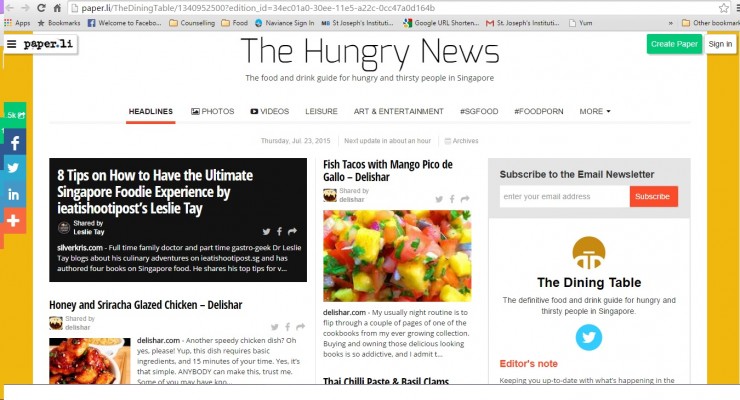Screenshot of a webpage from Hungry News featuring various sections like Headlines, Photos, Videos, Leisure, Art and Entertainment, SG Food, Food Porn, and more. The Headlines section is highlighted in red. On the left side of the page is a logo for paper.li, and on the right, there are buttons for "Create Paper" in a green rectangle and "Sign In" in a white rectangle. The body of the webpage shows numerous articles in gray font. The top article is titled "Eight Tips on How to Have the Ultimate Singapore Foodie Experience" by Ada Shoup's Leslie Tay, followed by a statement: "I eat is hoot. I post. I eat is hoot. I post - Leslie Tay." Other articles include recipes such as "Fish Tacos with Mango Pico de Gallo" and "Honey and Sriracha Glazed Chicken," both described as delicious.